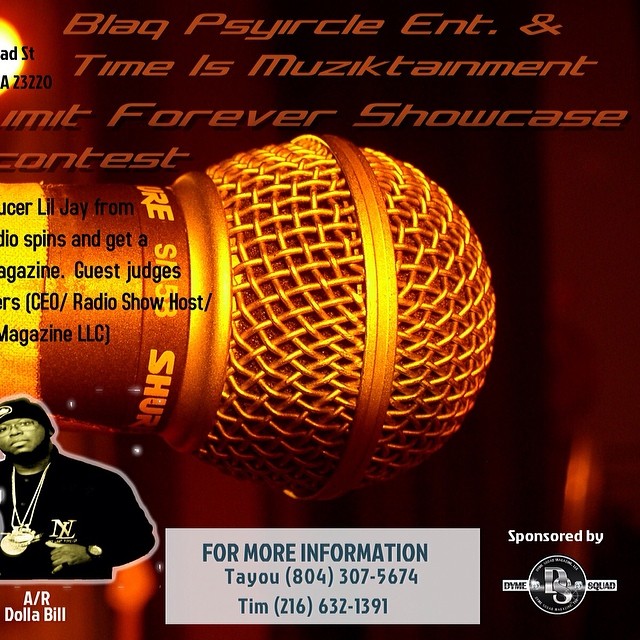This promotional flyer for a music show features a striking image with a black background and a golden-filtered Shure SM58 microphone pointing to the right. The text is centered, starting from the top with "Black Circle Entertainment and Time is Musictainment Summit Forever Showcase Contest." A prominent producer, Lil Jay from Radio Spins and Get a Magazine, is highlighted, alongside guest judges who are listed as CEO, radio show host, and magazine LLC.

On the flyer’s bottom left corner, there's a photo of an African-American man with several large gold chains and a black toboggan, identified as A.R. Dolla Bill. Towards the bottom right, the flyer states it's sponsored by Dime Squad. For further information, contact Taiyo at 804-307-5674 or Tim at 216-632-1391.